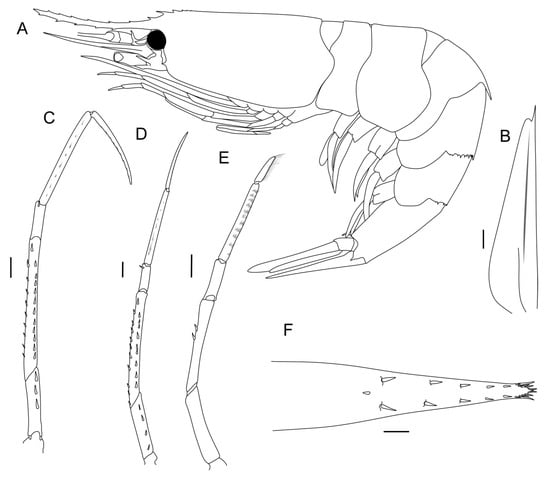The image is a detailed black and white illustration of a shrimp, presented in multiple views typically seen in an instruction manual or scientific diagram. At the top, there's a full-body view of the shrimp, facing left, with its tail bent into an oval shape. The shrimp has a distinctly shaded black eye. The illustration includes labels from A through F, designating different parts of the shrimp. The legs, jointed and segmented, are labeled C, D, and E, positioned on the left side of the image. The structure labeled B is on the right, with the tail section labeled F at the bottom. The drawing is entirely in black and white, against a white background, and features minimal shading with a few black spots marking specific details.